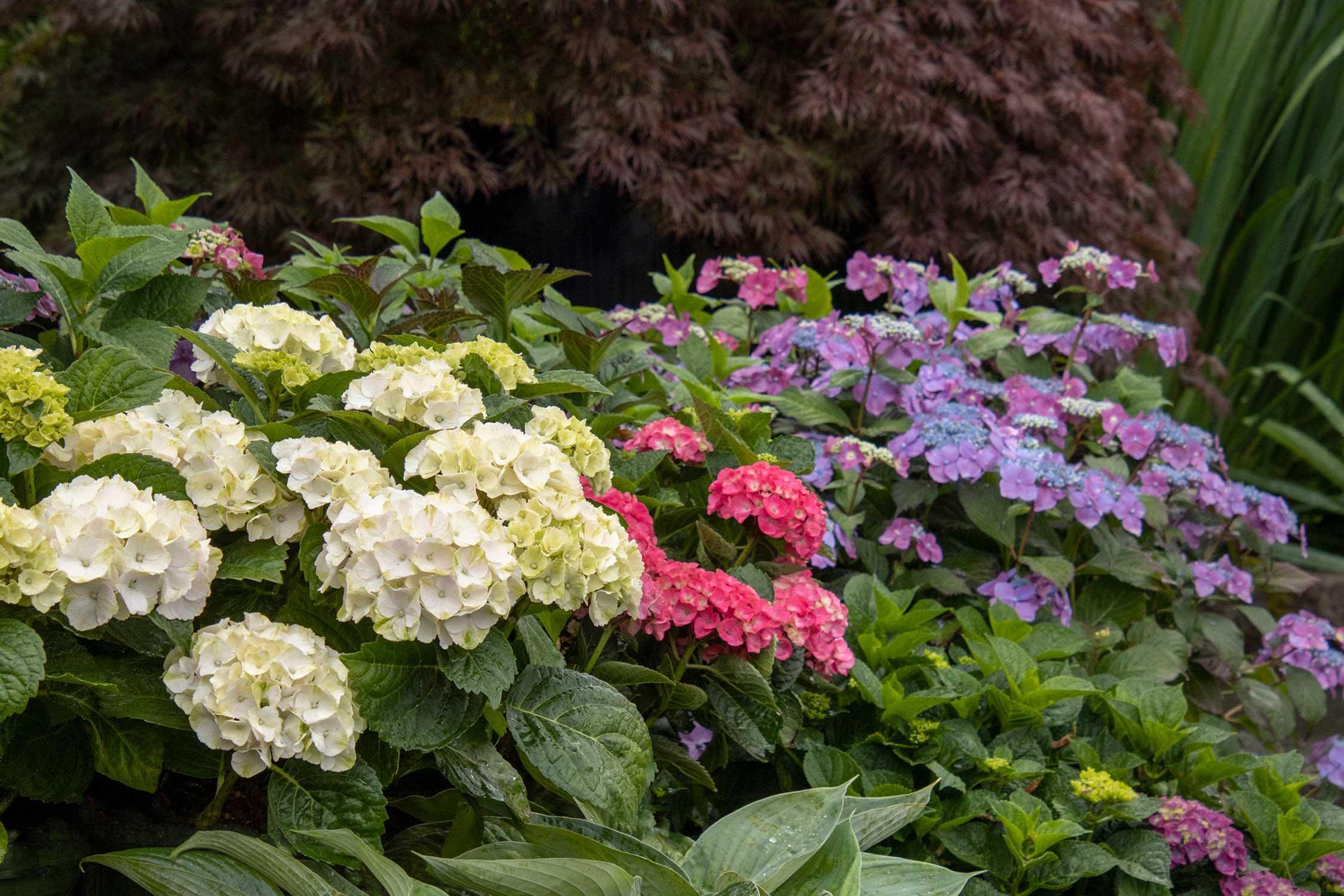This photograph captures a meticulously maintained garden in what appears to be summertime, showcasing a diverse array of flowering plants in vibrant, yet somewhat muted tones. Dominating the lower two-thirds of the image is a large, leafy bush adorned with clusters of hydrangeas in varying colors—white, pink, and purple, each exhibiting the characteristic cluster formation of the genus. Complementing these hydrangeas are some dark purplish flowers and a scattered appearance of lightly violet and pink-hued blooms, creating a harmonious, multi-colored display. The background displays a softly focused large bush and what appears to be Japanese maple with a mix of dark brown and auburn leaves. Additionally, there are tall green grasses and vegetation to the right of the frame, enhancing the lush, natural feel of the setting. The overall lighting suggests morning or a cloudy day, contributing to the vibrant yet subdued color palette of the scene.